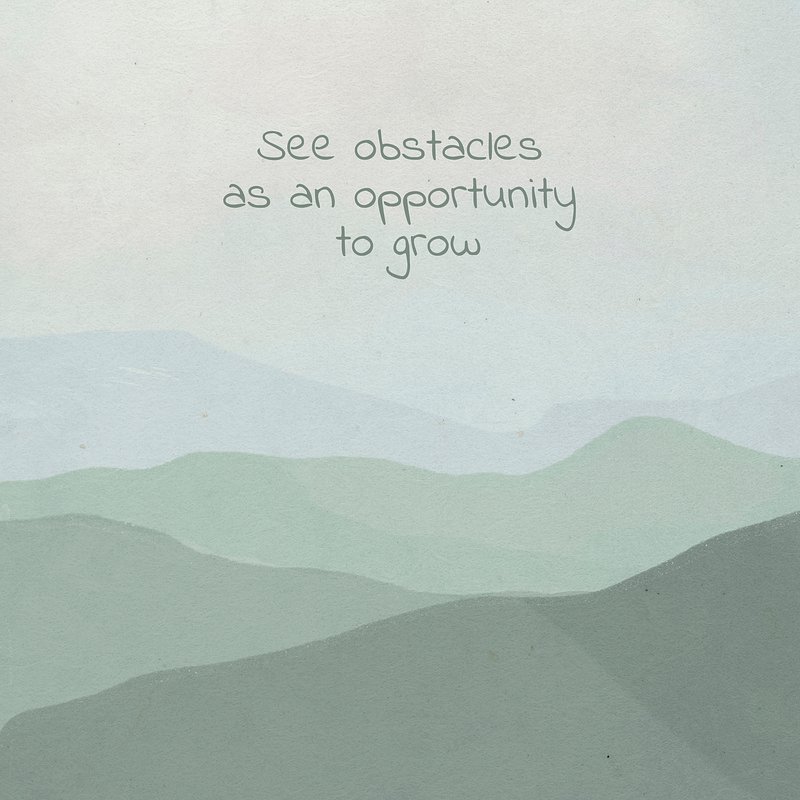**See Obstacles as an Opportunity to Grow**

This motivational poster features a serene and minimalist watercolor illustration of rolling hills and distant mountains, capturing the essence of perseverance and growth. At the bottom, the hills present an array of green hues, ranging from mossy to bluish-green and to grayish-green. The outlines are simple yet evoke depth, with each layer of hills blending seamlessly into the next. Moving towards the horizon, the hills gradually shift to lighter shades of blue, merging with a soft, off-white and pale gray sky at the top. The sky itself exudes a calm and peaceful ambiance, adding to the sense of tranquility.

Centered at the top of the image, the words "see obstacles as an opportunity to grow" appear in a dark green, understated font, devoid of capital letters, harmonizing with the overall simplicity and muted color palette of the artwork. This poster, with its elegant layers and comforting tones, inspires viewers to perceive challenges as pathways to personal development and tranquility.